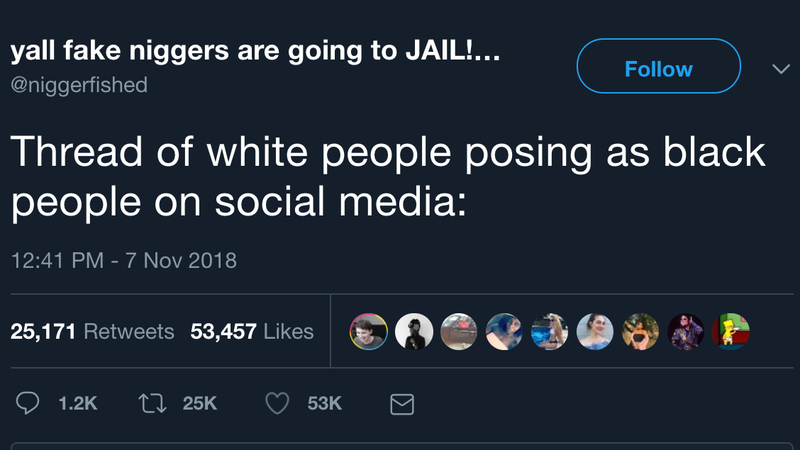The image depicts a screenshot from a social media site. The background is completely black with a bold white text at the top that states "yall fake n*****s are going to JAIL!!!" The word 'yall' is written without an apostrophe, and 'JAIL' is in all capital letters, followed by three periods. The user's name, displayed underneath, is "@n*****fished".

To the right, there's an outlined blue oval with the word "Follow" inside it, where the 'F' is capitalized. Below this, another line of white text begins with a capital 'T', saying "Thread of white people posing as black people on social media". The timestamp reads "12:41 p.m. 7 Nov 2018".

A separating line is then followed by the engagement metrics: "25,171 Retweets" and "53,457 Likes", both with capital letters. There are nine user profile image circles showing below this information. Further down, the comment section shows "1.2k" for comments, "25k" for retweets, "53k" for likes represented by hearts, and an envelope icon appears, indicating messages.

All information is formatted to convey a detailed and clear description of the screenshot.